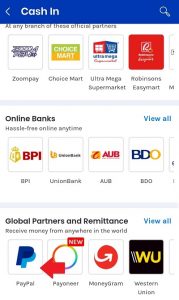This portrait-oriented screenshot, albeit blurry, appears to be from a cash transfer application. The top section features a header labeled "Cash In," suggesting it's a page dedicated to depositing money. In the upper right corner, there is a search bar for easy navigation. Just below it, the text reads "at any branch of these official partners," followed by four logos representing the partners: ZoomPay, ChoiceMart, Ultra Mega Supermarket, Robinson's, and Easy Mart.

A gray stripe demarcates the next section, which is titled "Online Banks," and promises "hassle-free, online anytime" banking. There is a blue link stating "view all." Under this section, the app lists partnered banks including BPI, Union Bank, AUB, and BDO.

Further down, another bold header announces "Global Partners and Remittance," with a blue "view all" link nearby. It claims that users can "receive money from anywhere in the world" via services like PayPal, an unspecified "Pay" service, MoneyGram, and Western Union, each accompanied by their respective icons.

Overall, the page appears to be geared towards offering various methods for users to cash in money, either via offline partners, online banks, or global remittance services, likely as a reward for completing offers, studies, or surveys.